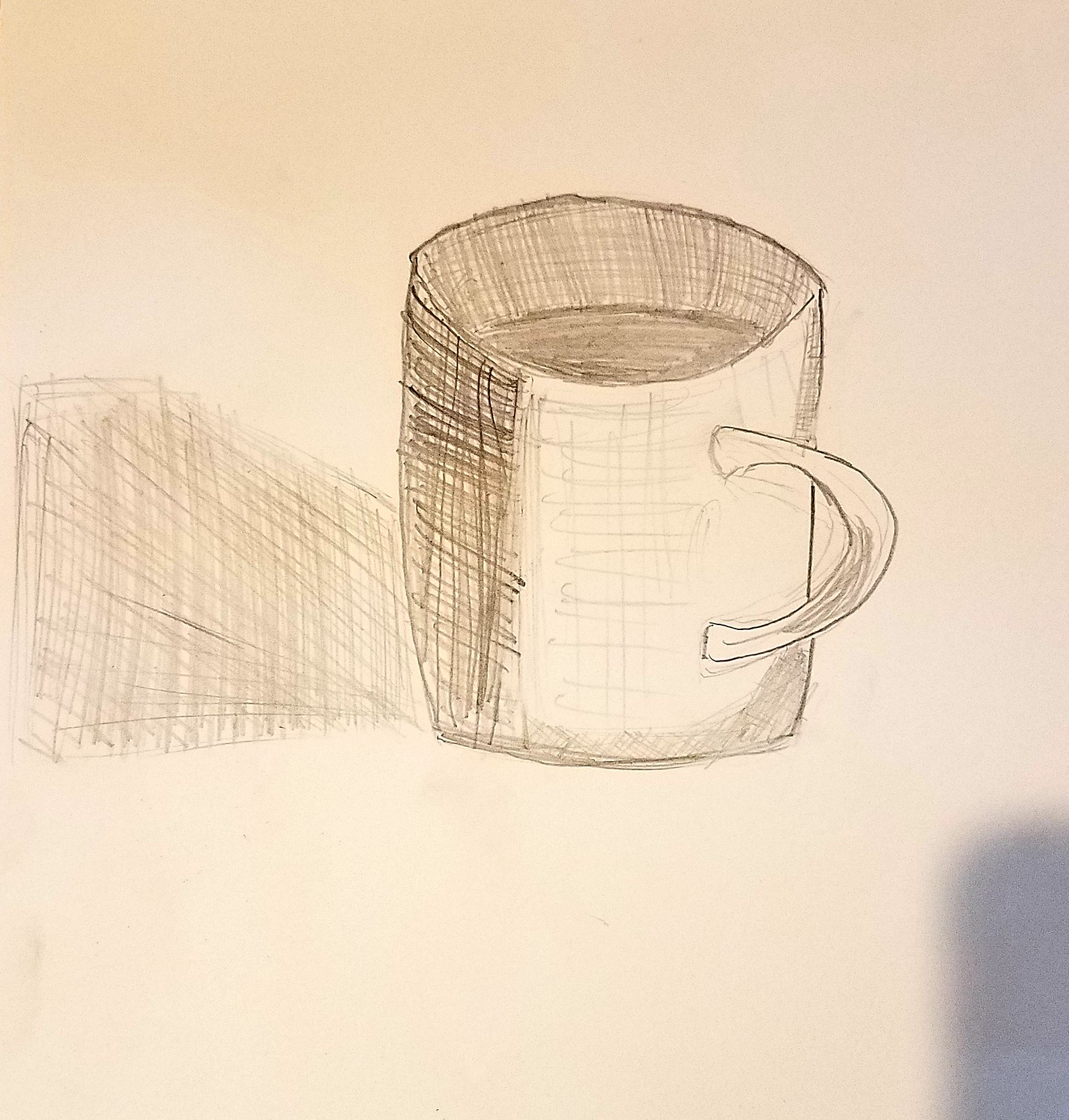This image displays a hand-drawn pencil sketch of a coffee mug on a white piece of paper. The mug, seen from a side view, features a rounded handle on the right and casts a pronounced shadow on its left, indicating the light source is on the right. The interior of the mug is shaded, suggesting it contains coffee. The drawing utilizes substantial line work, consisting of up-and-down or cross-hatching scribbles to depict shadows and depth, giving the mug a simple yet realistic appearance. In the bottom right corner of the image, there's a noticeable shadow that might be from a phone, implying the photo was taken from above. Despite its novice look, the drawing effectively captures the basic elements of a coffee mug in black and white pencil strokes.